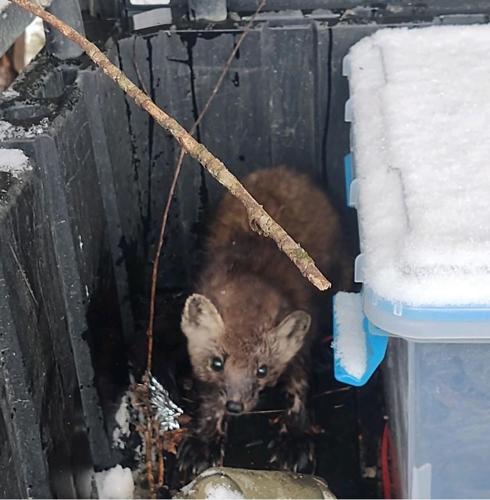The image shows a brown, raccoon-like animal with pointy ears, a black nose, and black eyes, appearing trapped in a black dumpster or small, fenced area. The animal is making direct eye contact with the camera, suggesting distress or curiosity. Surrounding the animal inside the dumpster are brown branches, some leaves, and a few pieces of trash. Notably, there is a clear Tupperware container with baby blue handles and red accents on its sides, topped with snow, to the right of the animal. The scene is set in a neutral-colored environment featuring shades of brown, white, gray, tan, and black, with only the Tupperware providing blue and red accents. The image appears to be a candid shot likely taken with a cell phone, characterized by its natural, unprofessional composition. There is no text or labeling in the image. A gray fence is visible in the background, adding to the sense of confinement. The overall setting suggests a daytime snow-filled environment with elements of melting snow and water.